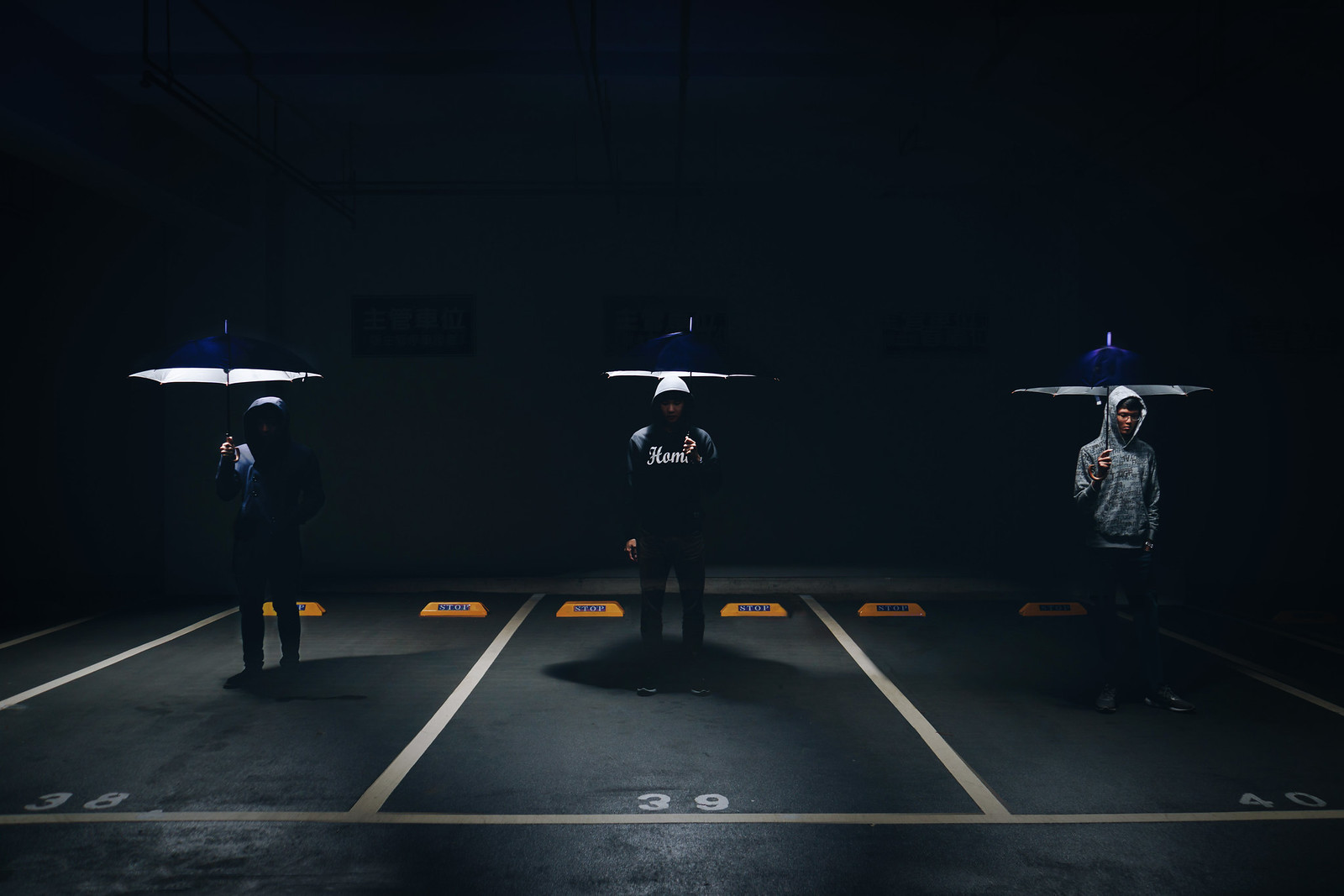In this dark, almost surreal nighttime photograph, three individuals stand in consecutively numbered parking spaces marked 38, 39, and 40, each delineated with white lines and ending in orange rectangular STOP signs on the ground. The setting appears to be an outdoor parking lot, shrouded in pitch-black darkness, which renders the figures starkly lit by the light built into their umbrellas. These umbrellas, held high above their heads, cast a downward glow, illuminating their hooded figures. Each person is wearing a hoodie with the hoods pulled up; the first on the left is clad in a darker hoodie, the middle individual sports a hoodie with a partially visible logo reading "H-O-M," while the third person on the right dons a lighter-colored, gray hoodie and glasses. All three umbrellas appear to be dark blue, enhancing the mysterious atmosphere. In the background, one can discern some indistinct Asian lettering on what looks like poster-style signs, adding an additional layer of enigma to the scene. The ground they stand on appears to be dark, perhaps asphalt or black-painted concrete, further accentuating the illuminated subjects in this artistically staged tableau that evokes a sense of contemplative isolation.